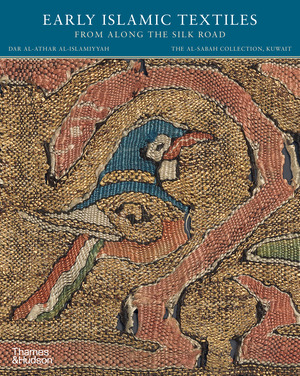The image depicts the cover of a book titled "Early Islamic Textiles from Along the Silk Road" by Dar al-Athar al-Islamiyyah from the Al-Sabah Collection in Kuwait, published by Thames and Hudson. The top of the cover features a blue border with the title inscribed in white text. Below, there is a detailed, earthy-toned textile image showcasing a bird with a red beak, a blue head, white area around the eyes, and a gold ring around its neck. Surrounding the bird, a snake in red coils intricately, the ensemble rendered in rich yellow textile. The detailed fabric design appears historical and meaningful. The publisher's name, Thames and Hudson, is located in the bottom left corner.